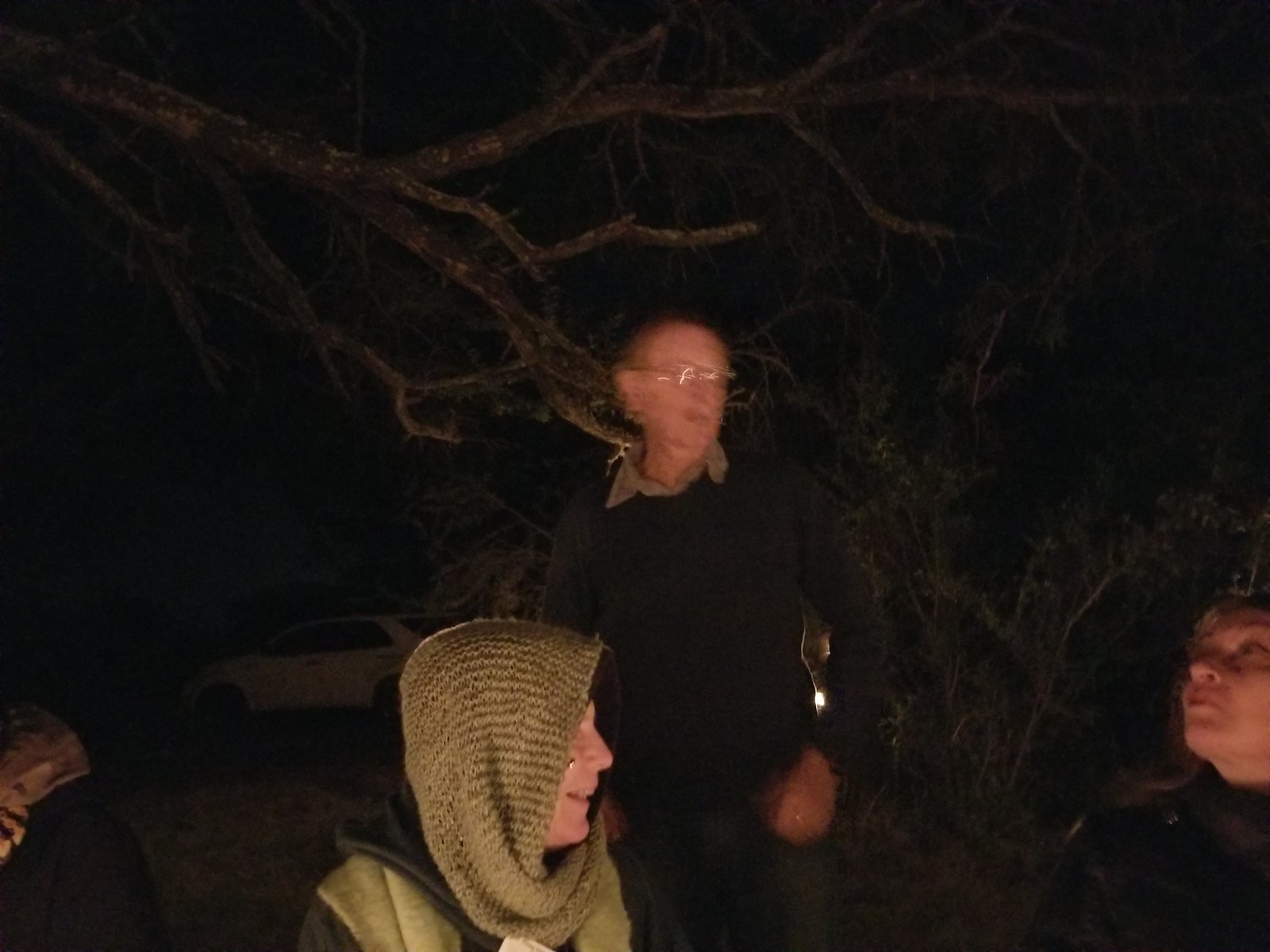In this photograph, taken in the dark with a predominantly black background, three individuals are prominently featured. 

To the left of the image is a shadowy outline of a white car, partially visible in the lower left corner. Above, a barren brown and black branch stretches across the top of the image, devoid of leaves. On the right-hand side, there is a faint shadow of some shrubs.

Standing prominently in the center is an older white man with glasses. He is dressed in a black sweater, from which a brown collar emerges. Below him, seated and captured from the shoulders up, is another person with white skin. This individual wears a green scarf wrapped around their head and a gray and black jacket. 

On the far right edge of the photograph is the third figure; only their face is visible as the top of their head is cut off. They have fair skin and appear to have blonde hair, accompanied by a black shirt.